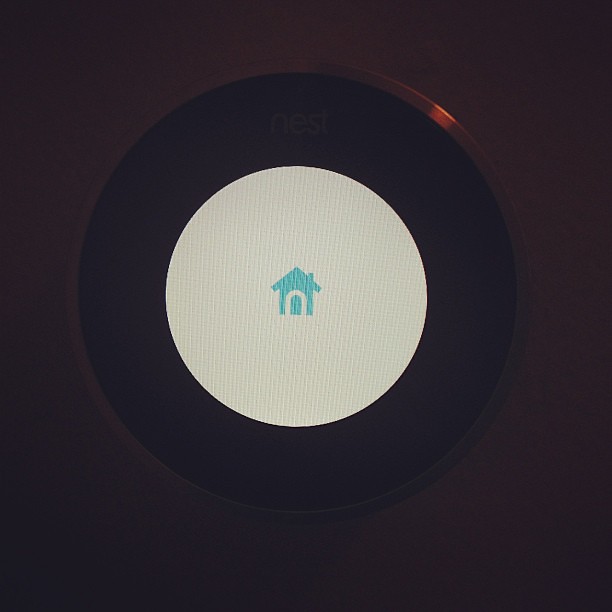Displayed is an image described as follows: It features a large, square object set against a stark black background, which appears smooth and textureless. The background subtly shifts in tones, with slight shadows and highlights adding depth and varying shades of black depending on the direction of the light.

Encircling the square object in the center is a rim that initially blends with the black background before transitioning into a deeper shade. Elements of red or orange punctuate the periphery, providing a hint of color variation. Directly within the central black area is a circular feature that evokes the appearance of a vinyl record, characterized by its pronounced thickness and deep black hue.

Prominently displayed on the upper section of this central black circle, in sleek grey letters, is the word "Nest" (N-E-S-T), identifiable as the logo of the popular home automation brand. Inside this circle lies a smaller, off-white inner circle adorned with fine, textured lines running in various directions, lending a tactile quality to the otherwise smooth surface.

At the very heart of this inner circle is a small blue house icon, emblematic of the Nest logo. This emblem adds a point of focus, grounding the composition and signifying the brand identity.